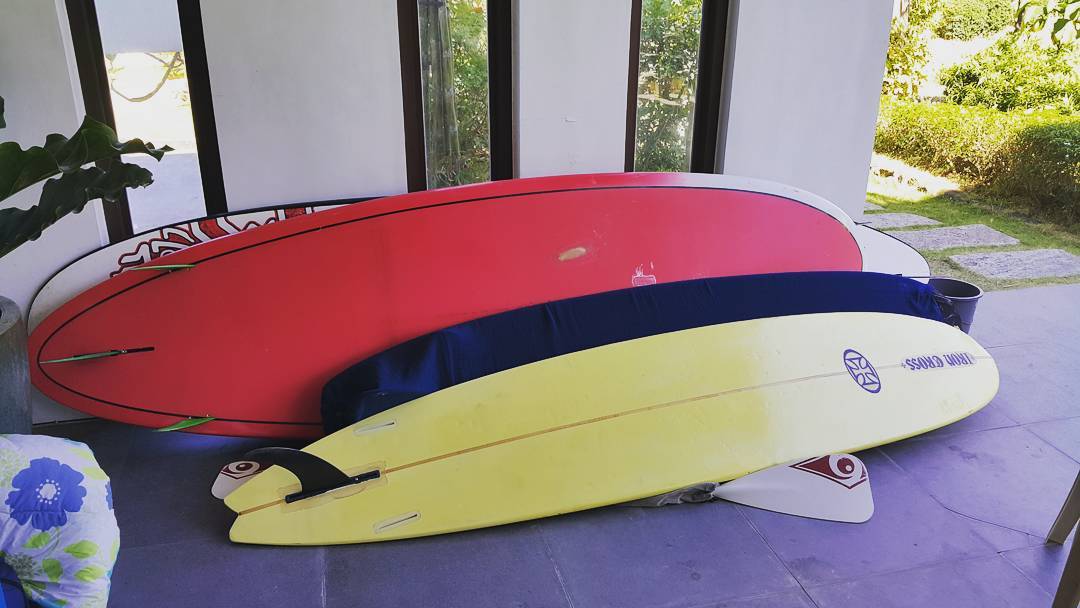This photograph captures a modest patio area outside a white-walled house with narrow, vertical windows reflecting nearby trees. Four surfboards of varying sizes are neatly leaning against the wall: a bright yellow surfboard at the front labeled "Iron Cross", followed by a navy blue surfboard wrapped in protective covering, a solid red surfboard with three visible fins, and partly obscured behind these, a white surfboard with a red and white floral pattern. The surfboards rest on a sophisticated, gray stone tile surface which contrasts with a nearby stone paver path that curves to the left, surrounded by well-maintained greenery and shrubbery. On the left side of the image, there's an inflatable or cushion-like object featuring blue and purple floral patterns. In the background, hints of a lush garden and potentially a cactus-like plant add a touch of nature to this otherwise structured and serene setup, suggesting a coastal vicinity.